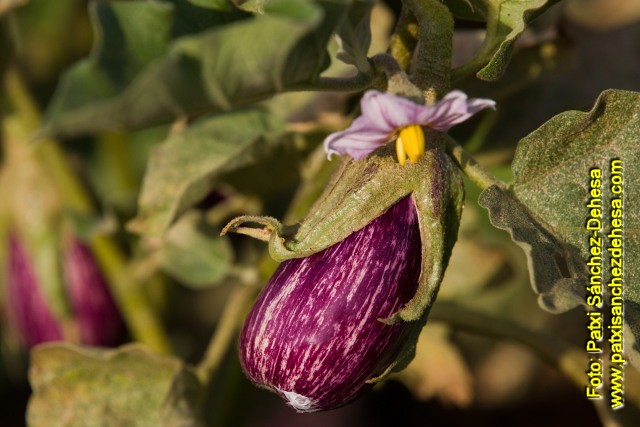This close-up photograph captures an emerging flower bud just starting to bloom from a green pod. Positioned centrally and stretching to the bottom middle of the image, the bud displays a blend of purple and white hues with a hint of yellow at the top. Encircling the budding flower are withered green leaves, adding texture and contrast. The image maintains sharp focus on the central flower, while the background fades into a blur of green foliage and distant purple pods, maintaining the emphasis on the main subject. On the right side of the photograph, yellow lettering running vertically reads "photo paxisanchez.deesa www.paxisanchezdeesa.com," suggesting the image is part of an advertisement. Additional leaves and branches adorn the left and right sides, with a clear, focused leaf branching off to the right, enhancing the composition of this botanical portrait.